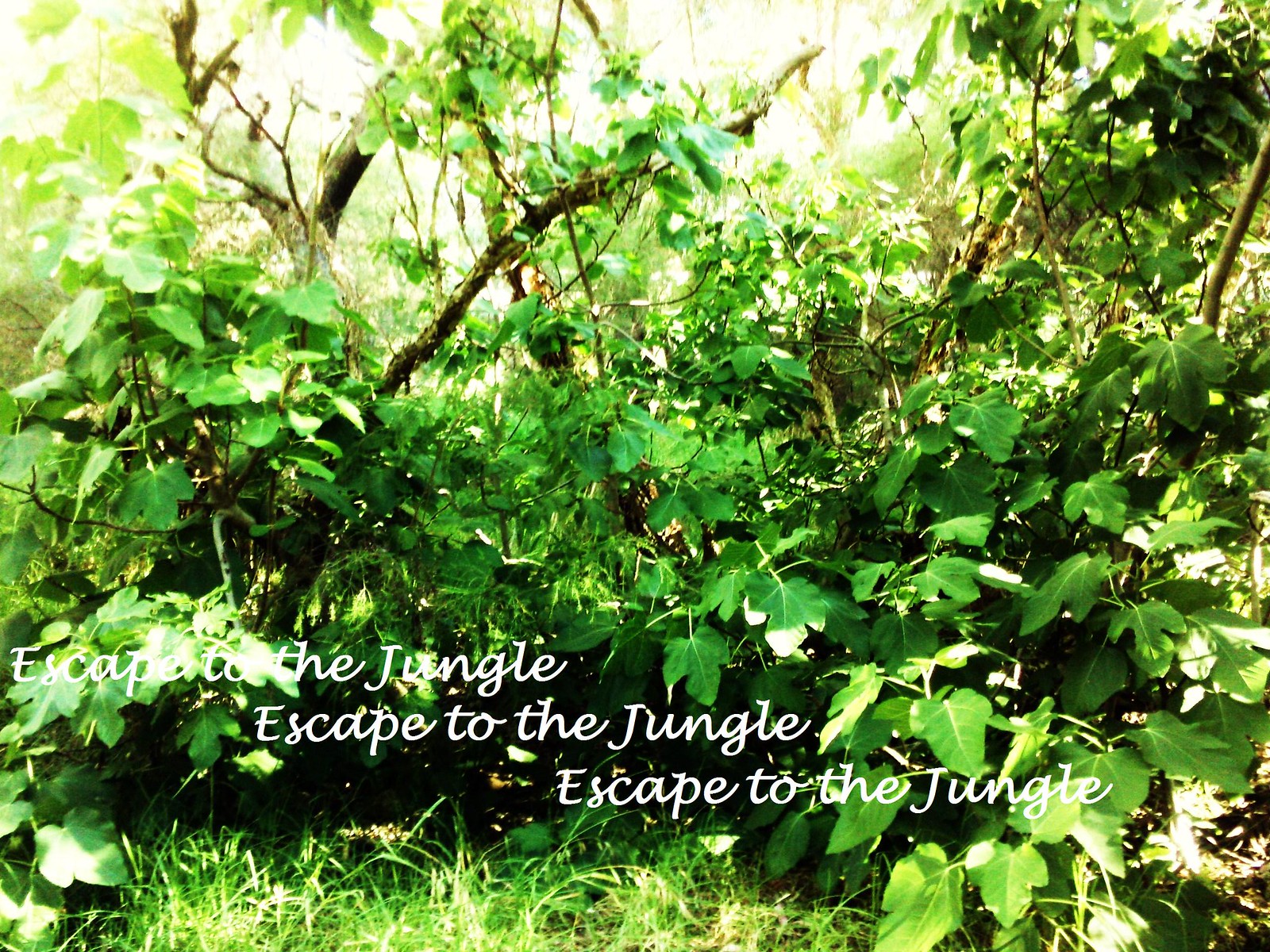The photograph, taken outside on a very sunny day, captures a vibrant, natural scene. Dominated by a lush green bush intermixed with vines, weeds, and small trees, the image portrays the diversity of plant life. Tall grass can be seen at the bottom, gradually blending into the dense foliage. Sunlight floods the scene, creating bright highlights on many leaves and causing the background to appear intensely bright. In the bottom left corner, large, thick leaves are prominently visible. The top right of the image also features a cluster of branches with leaves. Overlaying the bottom of the photo, in white cursive font, the phrase “Escape to the Jungle” is repeated three times in descending order, mimicking a step-like pattern as it partially merges with the sunlit background.